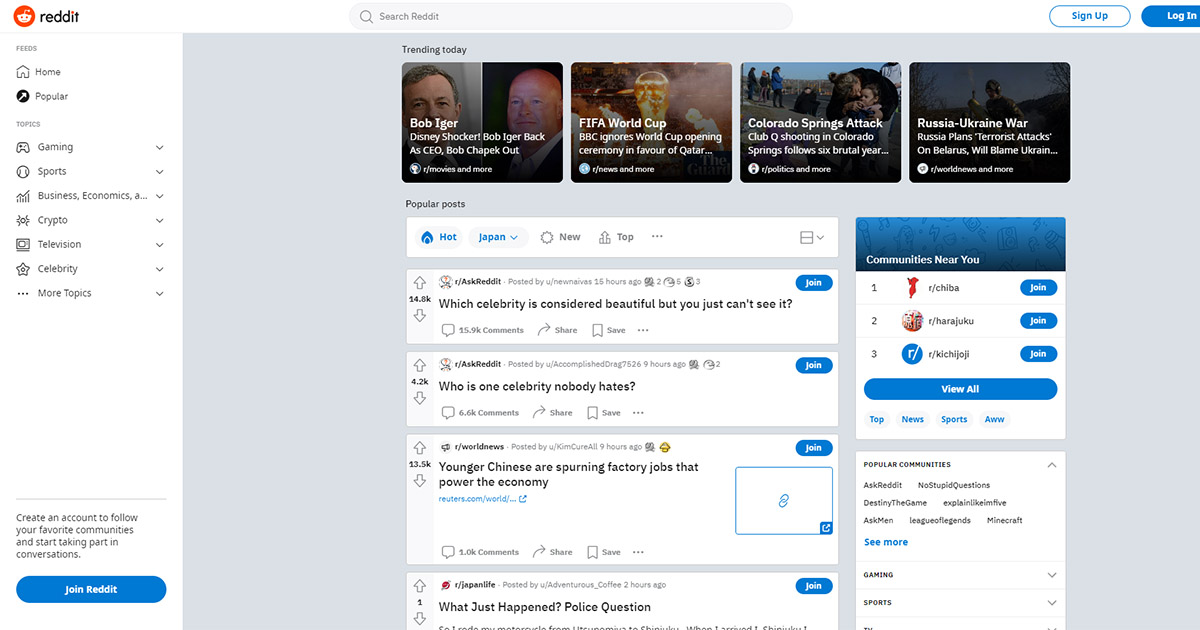This is an image that captures a screenshot from the Reddit website, displayed on a horizontally rectangular frame. 

In the upper left corner, the distinctive Reddit logo is visible. Directly centered across from the logo is the search bar labeled "Search Reddit." To the far right, slightly cut off, are the "Sign Up" and "Login" buttons, with the "Login" button's right edge cropped out of the frame.

On the left side of the image, there is a vertically rectangular white background housing various feed options. Under this section, we find tabs labeled "Home" and "Popular," followed by several categorized topics. Each topic listing features a drop-down arrow for more specific search options and includes categories such as "Gaming," "Sports," "Business," "Economics," "Crypto," "Television," "Celebrity," and a final category labeled "More Topics." At the very bottom of this section, a prominent blue "Join Reddit" button is displayed.

The remainder of the frame displays a light gray background. Centered in this section, the headline "Trending Today" appears at the top, above four side-by-side images. Each image has a headline corresponding to trending topics: "Bob Iger," "FIFA World Cup," "Colorado Springs Attack," and "Russia-Ukraine War."

Below these trending topics, there is a listing of popular posts and questions, featuring headlines like "Which celebrity is considered beautiful but you just can't see it?", "Who is one celebrity nobody hates?", "Younger Chinese are spurning factory jobs that power the economy," and "What just happened? Police question...".